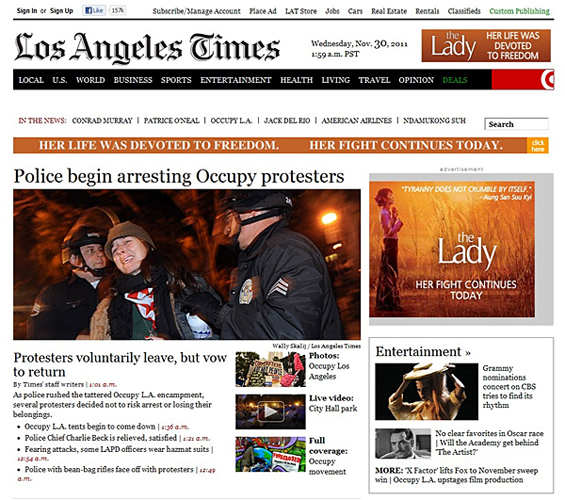This is a detailed descriptive caption for the image mentioned:

The image appears to be a desktop screenshot of the Los Angeles Times website. In the top left corner, there are options for signing in or signing up, accompanied by a rectangular blue button indicating Facebook-like engagement with '50%' or '157K likes'. To the right, options include 'Subscribe/Manage Account', 'Place Ad', 'Flat Store', 'Jobs', 'Cars', 'Real Estate', 'Rentals', 'Classifieds', and 'Custom Publishing' in green text. A black line separates this toolbar from the main content.

The header of the page prominently features the title 'Los Angeles Times' in a classic Romantic style of font. The timestamp below reads 'Wednesday, November 30, 2011, 1:59 AM PST'. Further to the right, an advertisement with a dark orange background states "Lady, her life was devoted to freedom".

Beneath the header is a navigational bar with tabs labeled 'Local', 'US', 'World', 'Business', 'Sports', 'Entertainment', 'Health', 'Living', 'Travel', 'Opinion', and 'Deals' – the latter in green lettering. This navigational strip has a black background with all other text in white. To the right of 'Deals' is a red rectangular section with a half-target logo on the far right.

The featured headline reads, "Police begin arresting Occupy protesters," accompanied by a photograph of police officers flagging a protester. The scene appears to be captured at night, illuminated by artificial light, with silhouetted trees visible in the background.